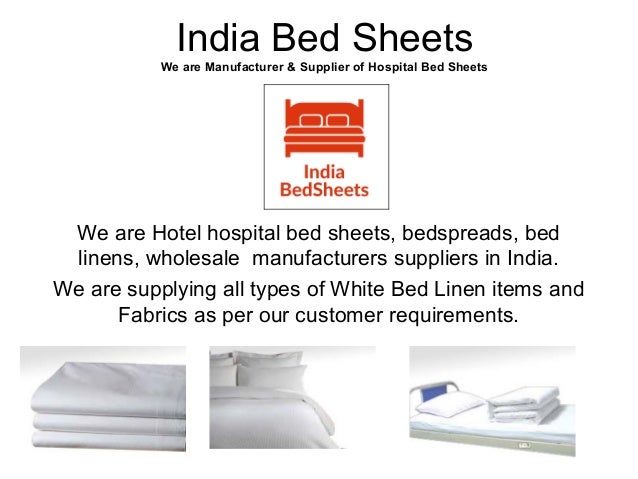The advertisement image for India Bed Sheets features a clean, white background with text and visuals organized in a clear manner. At the top, the brand name "India Bed Sheets" is displayed in Arial font, followed by a statement declaring "We are manufacturer and supplier of hospital bed sheets." Below this text, the brand's logo is displayed within a red square, showcasing an orange icon of a double bed with two pillows and a blanket. Beneath the logo, additional text details, "We are hotel, hospital bed sheets, bed spreads, bed linens, wholesale manufacturers, suppliers in India. We are supplying all types of white bed linen items and fabrics as per our customer requirements."

At the bottom of the image, three photos are arranged from left to right. The first photo shows neatly folded and stacked bed sheets. The middle photo features a well-made, plump bed adorned with white sheets and pillows. The last photo displays a more utilitarian bed, which could be interpreted as a hospital bed, with some folded sheets placed on top. The overall bright and minimalist design highlights the different types of bed linens available, reinforcing the brand's expertise and range in supplying high-quality, white bed linen items.